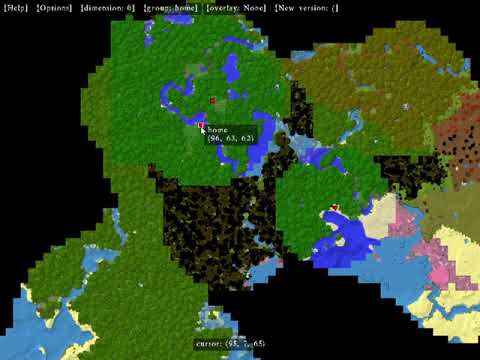The image resembles a two-dimensional, pixelized video game map viewed from an aerial perspective. Dominated by shades of green, the map features various colors indicating different terrain and elements: blue regions suggest rivers and lakes, dark green and black areas denote dense forests, and there are scattered patches of pink, yellow, brown, beige, and red. The background is solid black, potentially representing uncharted or deep-water zones. In the center, a red structure is highlighted by a cursor, labeled "home." At the top right, there is readable text "help" and "options," with other less legible words indicating game settings and version details. Additionally, there are some coordinates at the bottom of the screen, albeit blurred.